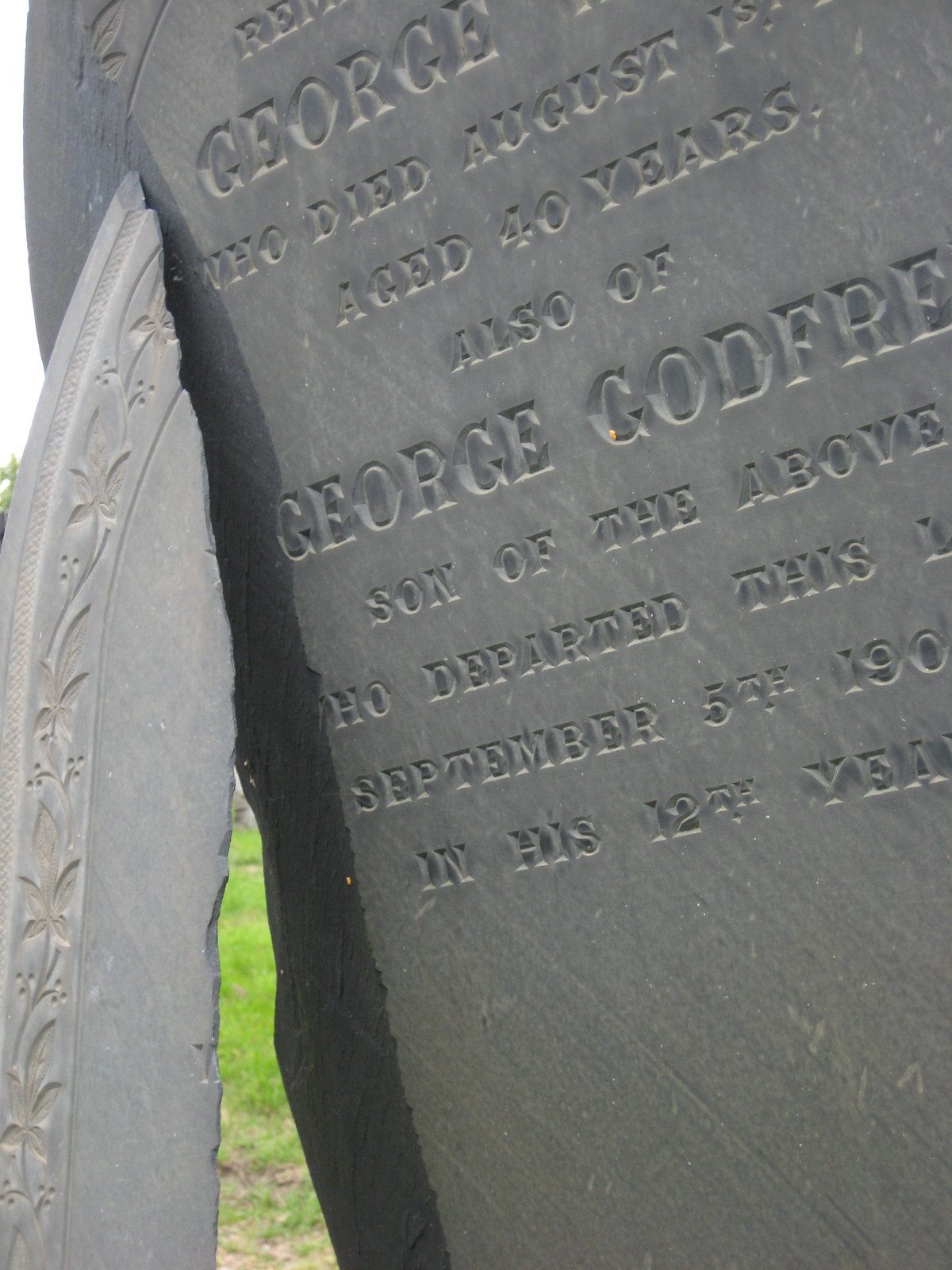This close-up photograph vividly captures an old and slightly damaged gravestone, prominently filling the frame. The dark gray, thick gravestone features a rectangular body with a round top and an ornate floral border. A large chunk appears broken off the left side, leaning against the main stone. This break exposes a small patch of grass at the bottom of the image. Despite its age—over a century old— the gravestone remains in relatively good condition with no signs of moss, hinting at smooth, durable slate material. The embossed text is partially visible and reveals a poignant history: "George, who died August 1st, aged 40 years," alongside "George Godfrey, son of the above, who departed this life September 5th, 19--, in his 12th year." The serif-style engraving, all in capital letters, highlights the names with a larger font, adding solemnity to the memorial.